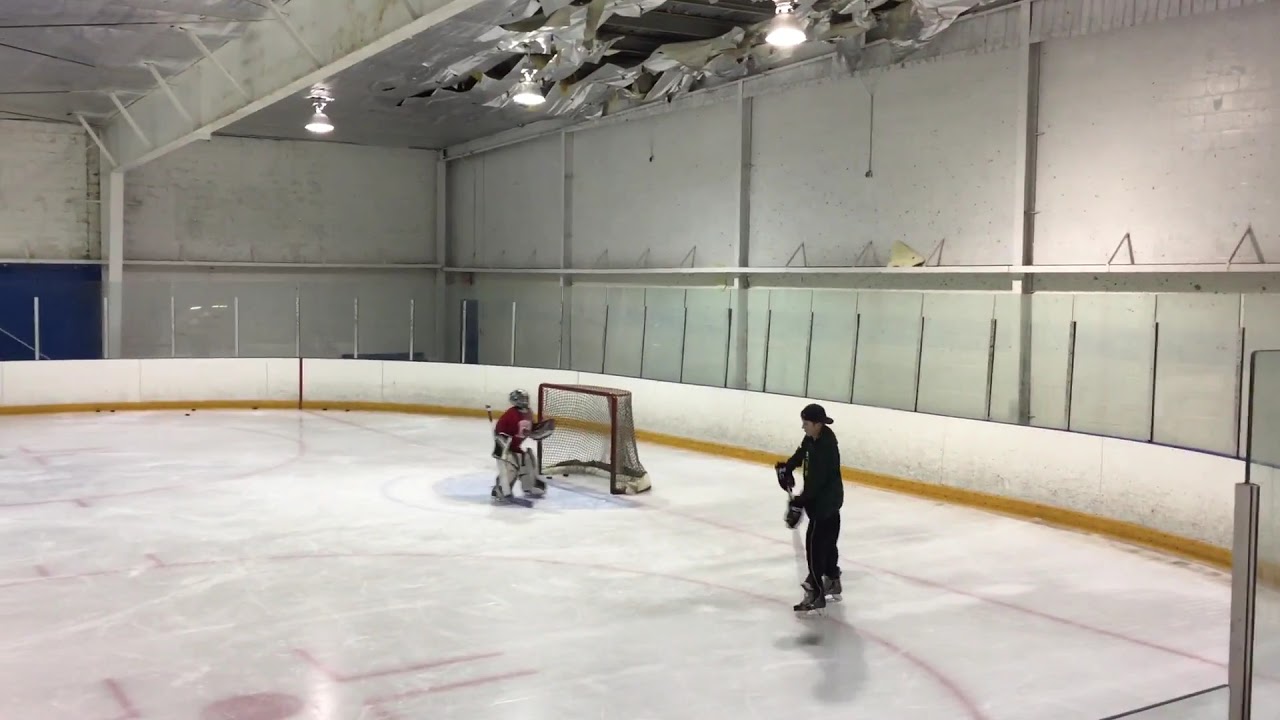In a tranquil, empty hockey stadium, captured with photographic precision, the scene showcases a training session. The white ice rink, marked with red face-off circles and bordered by white walls, provides a stark, clean environment. To the right, the goalie, clad in a red jersey, white pants, and a white helmet, stands poised with pads and stick, facing a man in black. This man, wearing black skates and a backwards black baseball cap, is armed with a hockey stick, appearing ready to engage in practice. They are positioned near the goal post, partly framed by a white wall with sections of blue doors. Overhead, three bright lights illuminate the rink, casting a spotlight on the duo. The ceiling shows signs of wear with peeling paper, adding a touch of imperfection to the otherwise pristine rink. The atmosphere is calm and focused, devoid of any audience, encapsulating a moment of quiet preparation.